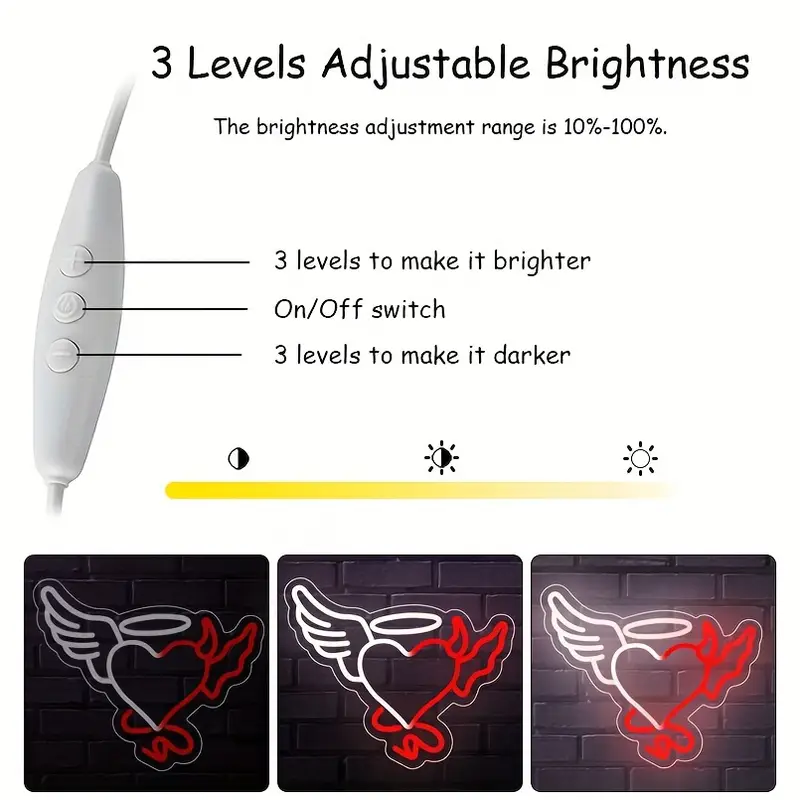The top image showcases a white control switch designed for brightness adjustment. The switch allows for three levels of brightness, with an adjustment range from 10% to 100%. The switch also features an on/off function and gauges to indicate various brightness levels.

Below the control switch, there are three separate images arranged horizontally, depicting a gray brick wall adorned with an illuminated, neon-style heart sign. The heart is artistically divided into two contrasting halves. The left side is white, featuring an angel wing extending from it and a halo hovering above. The right half of the heart glows red, adorned with a devil horn, wing, and tail extending from the bottom. 

The three images show varying brightness levels achieved using the control switch. The image on the far left is the darkest, portraying the heart sign with minimal illumination. The middle image is moderately brighter, providing a clearer view of the details. The rightmost image is the brightest, with vibrant lighting that fully highlights the intricate angelic and demonic features of the heart sign. This sequence elegantly demonstrates the adjustable brightness capabilities of the control switch.